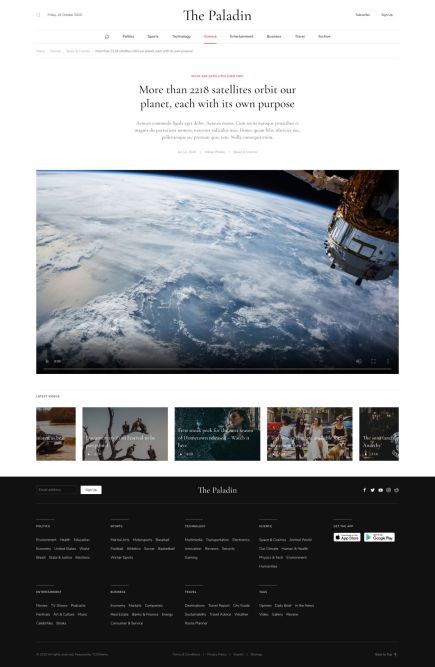The web page of "The Paladin" online newspaper is prominently displayed against a clean, white background. At the top center, in bold letters, reads the title "The Paladin." This is flanked by some unreadable information in the top left and top right corners, contributing to the typical layout of a news site.

Below the title, there are eight clickable sections, each leading to different parts of the newspaper. The text is mostly indistinct except for the one on the far right labeled "Archive."

Spanning the width of the page, just beneath this navigation bar, is a line of red text, which is illegible, followed by a large, striking headline in black typeface that reads, "More than 2,218 satellites orbit our planet, each with its own purpose."

A detailed, prominently positioned photograph follows this headline. It's a stunning satellite view of Earth, focusing on a partial view of the planet's surface. The top right portion of this image is black, representing the vastness of space, and prominently features a satellite. The satellite has a brown top with silver metallic rings below, occupying the top half of the top right corner of the photograph.

Beneath the primary photograph, there are five smaller rectangular images arranged horizontally, each symbolizing different articles with accompanying photos. These images depict various scenes including individual portraits, outdoor settings, and birds perched on trees.

Further down the page, a large black rectangle rests, emblazoned with "The Paladin" in white type. This area contains eight more sections for additional information. However, the text here is also blurry and undecipherable. To the right of this section, the page indicates it accepts payments via Google Pay and Apple services.